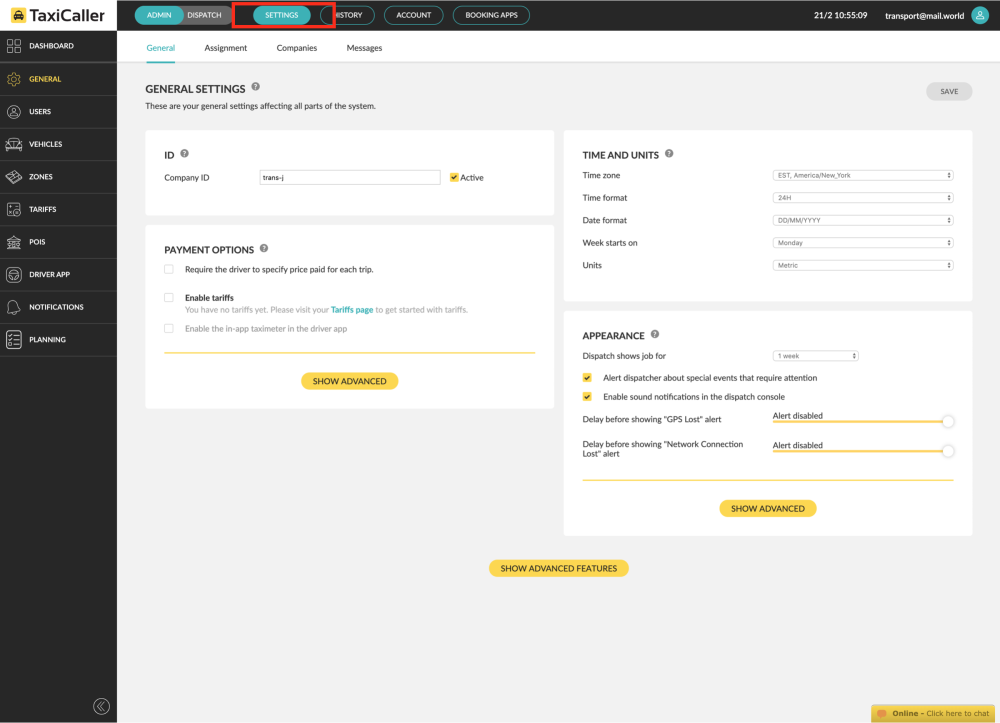This image depicts a section of a website interface created by Taxi Caller. The interface features a prominent yellow box with an icon of a taxi inside it. On the left, a vertical black navigation bar lists various sections including "Dashboard," "General," "Users," "Vehicles," "Zones," "Tariffs," "PC something," "Notifications," and what seems to be "Planning."

At the top of the interface, there is a horizontal black bar with options labeled "Settings," "Account," and "Booking Apps." The content within the main section of the website includes informational text such as "Temporal, World." Beneath this, a section titled "General Settings" indicates that these settings affect all parts of the system. This section details options like an ID field, an "Active" status, and "Payment Options." Users can enable tariffs, set time and date formats, choose when the week starts, and select units of measurement.

Further down, the "Appearance" section provides customization options like "Dispatch Shows Job 4," "Alert Dispatcher," "Enable Good Notifications in the Dispatch Capsule," and more. There is a noticeable yellow bar labeled "Show Advanced," which, when clicked, presumably reveals advanced settings. At the very bottom right corner, there is another yellow bar instructing users to "Click Here to Check Online."

Overall, the interface looks organized and user-friendly, with clear sections and highlighted options to streamline the management of taxi services.